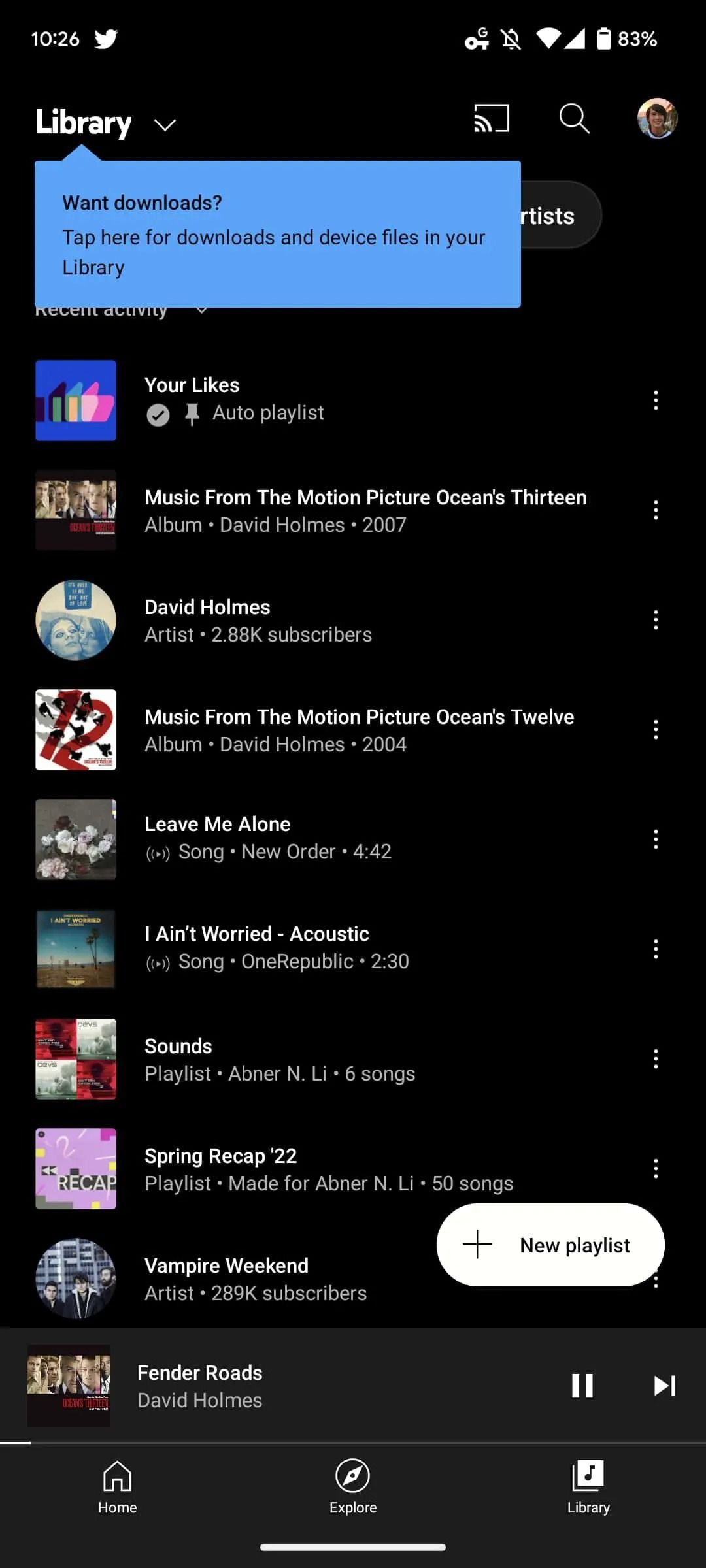This image is a detailed screenshot of a music application running on an Android device. In the top-left corner, the device time is displayed as 10:26 AM, accompanied by a Twitter icon. On the top-right, several icons are visible: a lock/key symbol, crossed-out notification bell, full Wi-Fi signal, full cellular signal bars, and an 83% battery level.

At the bottom of the screen, the library section is visible, with a blue disclaimer prompt indicating "Tap here for downloads and device files in your library." Adjacent to this is a TV icon with a Wi-Fi signal, showing that content is being cast to another device. There is also a search bar and a profile picture icon on the right side of the header.

Below the disclaimer, a series of songs and playlists are listed, each accompanied by album artwork on the left:

1. **Your Likes** (auto-playlist) - Displayed with a thumbs-up icon.
2. **Music from the Motion Picture, Ocean's 13** - Album by David Holmes (2007), featuring 2.88K subscribers.
3. **Music from the Motion Picture, Ocean's 12** - Album by David Holmes (2004).
4. **Leave Me Alone** - Song by New Order, duration 4:42.
5. **I Ain't Worried (Acoustic)** - Song by OneRepublic, duration 2:30.
6. **Sounds** - Playlist by Abner N. Lee, containing six songs.
7. **Spring Recap 2022** - Playlist made for Abner N. Lee, featuring 50 songs.
8. **Vampire Weekend** - Artist with 2.88K subscribers.

At the very bottom, the currently playing song is "Fender Rhodes" by David Holmes. The player controls are also visible, with options for "Home," "Explore," and "Library" at the bottom of the screen.

This comprehensive screenshot provides an overview of the user interface, currently available music content, and active features on the music application.